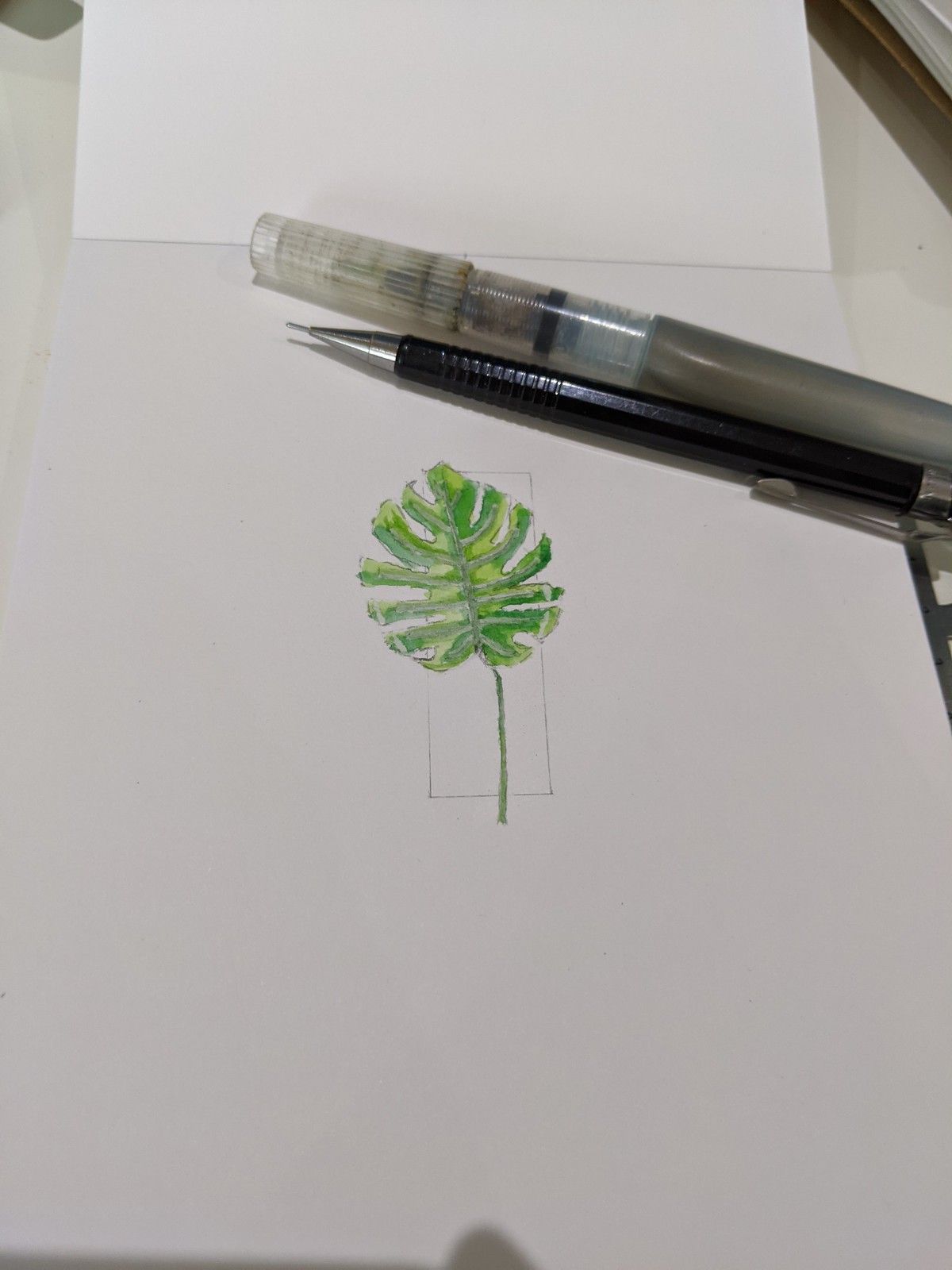A white sheet of paper, folded, showcases a detailed drawing. The interior is stark white, contrasting with various writing instruments scattered around: a gray pen with a red cap, a black pen with a silver cap on the left, alongside a collection of pencils and pens. These items are repeatedly placed—pens and pencils alternating in a meticulous arrangement.

The focal point of the drawing is a green leaf with a stem, framed by a black rectangle. White and green leaves are interspersed throughout, creating a balanced spread across the left and right of the paper. Subtle shadowing is present at both the top and bottom, enhancing the depth of the illustration.

In the top-right corner, alongside the main drawing, are two more writing implements—a pen and a pencil, contributing to the slightly dark ambiance of the image. The overall composition blends structured chaos with organic elements, producing a compelling visual story.